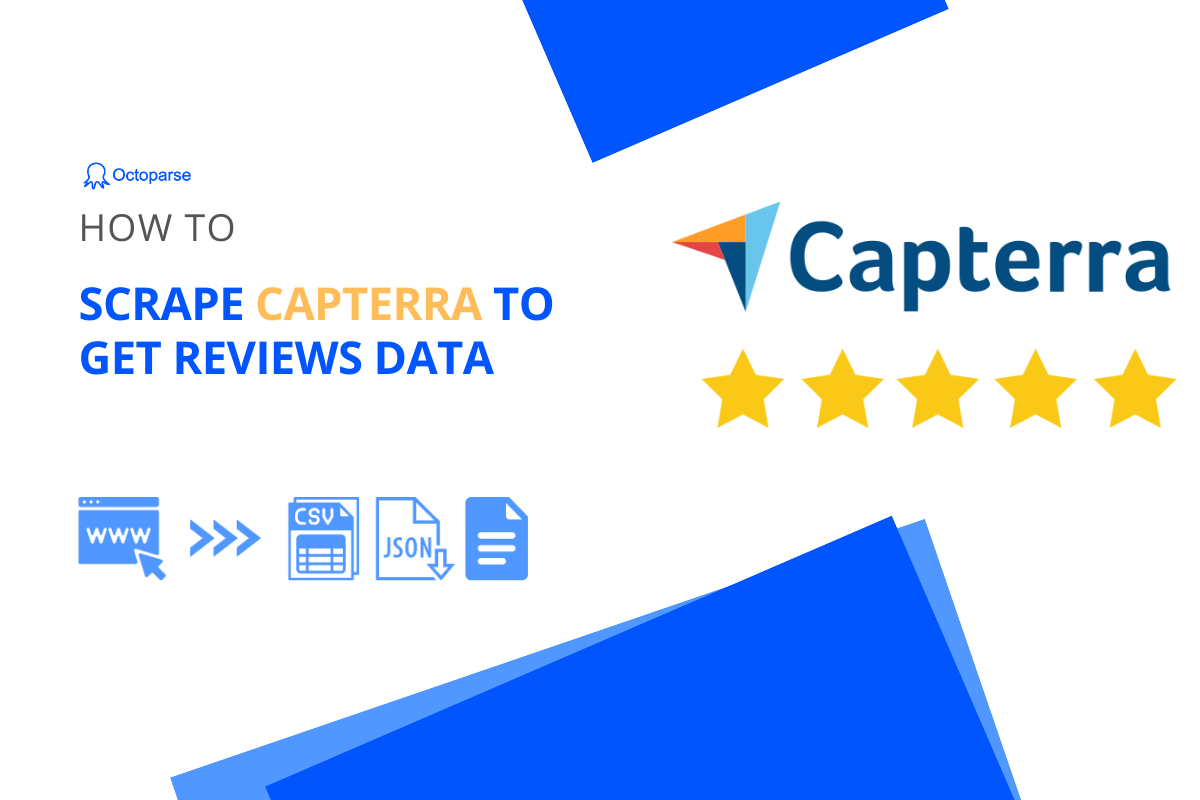This image is a detailed screenshot either from a webpage or an app. Dominated by a large white rectangle, the design features blue triangles at both the top and bottom for aesthetic appeal. In the upper left corner, the word "Octoparse" is prominently displayed. The title, "How to Scrape Capterra to Get Reviews Data," is clearly presented, with specific textual emphasis: "Scrape" and "to Get Reviews Data" are in blue, while "Capterra" is in yellow.

To the right of the title, there's a multicolored triangle icon adjacent to the word "Capterra" in blue letters, with five yellow stars positioned below it, likely emphasizing a review rating. Below the main header, there is a string of symbols beginning with "www" followed by a small arrow, and a sequence of three right-pointing arrowheads. Further to the right, there are abbreviations "CSV" on a blue paper icon and "JSON" on a white paper icon, accompanied by another icon of blue paper. This assortment of elements likely represents different data formats available for use.